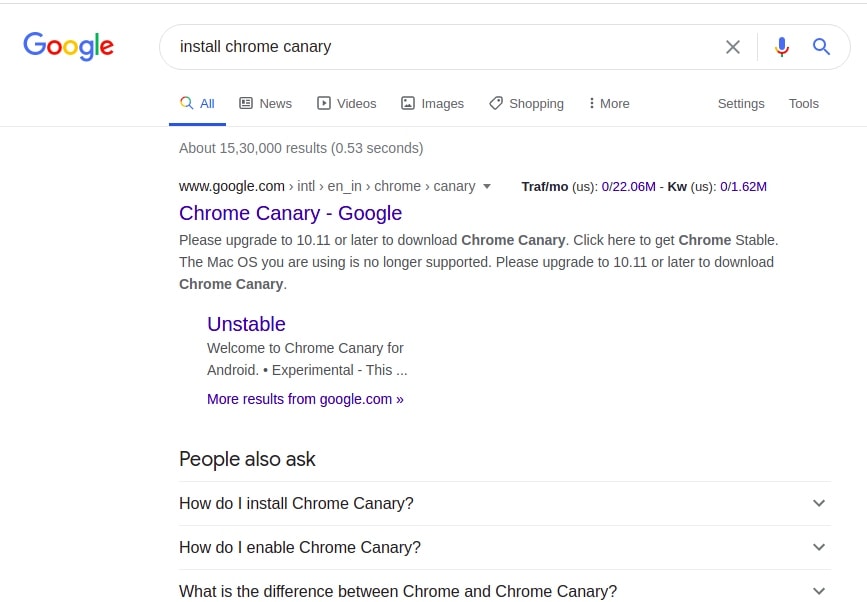This desktop screenshot features a detailed view of a Google search page. The browser and operating system details are omitted, with only the Google website interface visible. The user has conducted a search for "install Chrome Canary." The search interface displays typical Google search options such as "All," "News," "Videos," "Images," "Shopping," "More," "Settings," and "Tools," with "All" currently selected.

The search results indicate approximately 15,300,000 results, displayed within 0.53 seconds, although the figure is inaccurately formatted with commas in the wrong place ("15,000,000" instead of the likely correct "1,530,000" or "15,300,000").

The first search result is a URL: www.google.com, followed by a trailing path that includes I, an arrow (→), I-N-T-L, an arrow (→), E-N slash (/) I-N arrow (→) Chrome arrow (→) Canary, and ends with seemingly nonsensical characters and terms such as T-R-A-F slash (/) M-O-U-S, and others.

The main result is a notice stating "Chrome Canary - Google: Please upgrade to 10.11 or later to download Chrome Canary. Click here to get Chrome Stable. The macOS you are using is no longer supported. Please upgrade to 10.11 or later to download Chrome Canary." Below this, there is another link labeled "Unstable," introducing Chrome Canary for Android experimental purposes, inviting the user to explore further.

Footnotes under the main search results include suggested follow-up links and queries like:
- "How do I install Chrome Canary?"
- "How do I enable Chrome Canary?"
- "What's the difference between Chrome and Chrome Canary?"

This detailed search interface captures the precise information displayed and suggests the actions a user might take based on their search.